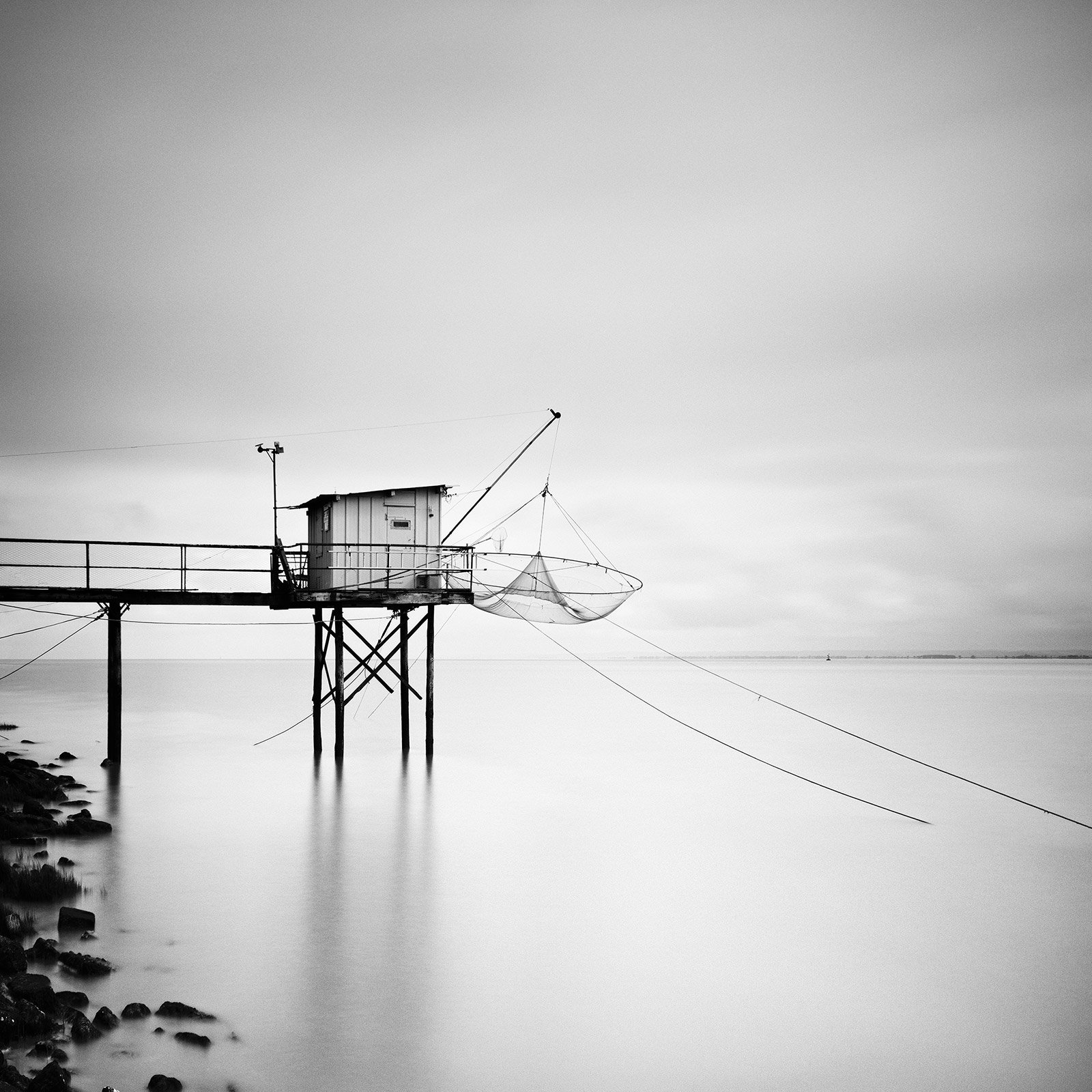This evocative black-and-white photograph captures a serene scene of a pier jutting out into a vast expanse of water, blending seamlessly with the horizon where the sky and water meet. The pier, adorned with long shadows, supports a small white structure with a flat roof and line patterns adorning its exterior. To the left of this building stands a lamppost, accompanied by a crane-like contraption from which a net dangles, suggesting basic fishing activities. Multiple fishing lines extend from the pier into the reflective, light gray water. Below this setup, the shallow water reveals a collection of black rocks and patches of grass in the bottom left corner, adding depth and texture to the image. The photograph exudes a dark and atmospheric tone, enhanced by the cloud-laden sky and the interplay of light and shadows across the scene.